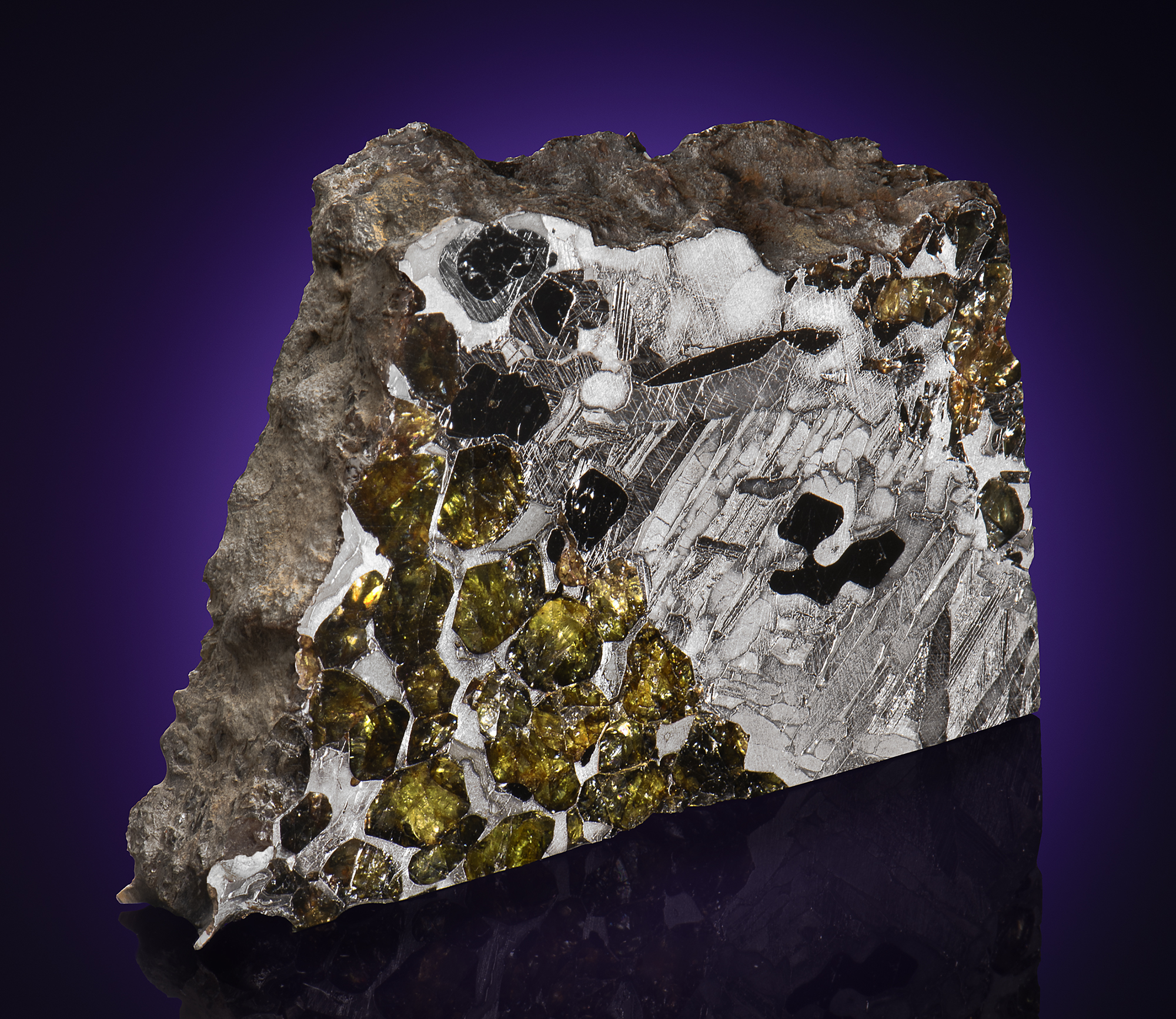The image showcases a trapezoid-shaped geode rock that has been finely sliced to reveal its intricate and colorful interior. The external edges of the stone are rough, gray, and dusty, contrasting sharply with the glossy, glass-like surface of the exposed face. This visible face is predominantly white with shattered, glassy inclusions extending from the lower right to the upper left corner. Embedded within this white substrate are sparkling yellow crystals concentrated in the lower left corner and extending towards the center, as well as in the upper right corner. A few black crystals are also scattered throughout. The rock slice is displayed on a reflective, dark purple or indigo surface, enhancing the vibrant and intricate details of the crystalline formations inside the stone. There's no text in the image, just the mesmerizing interplay of natural mineral formations.